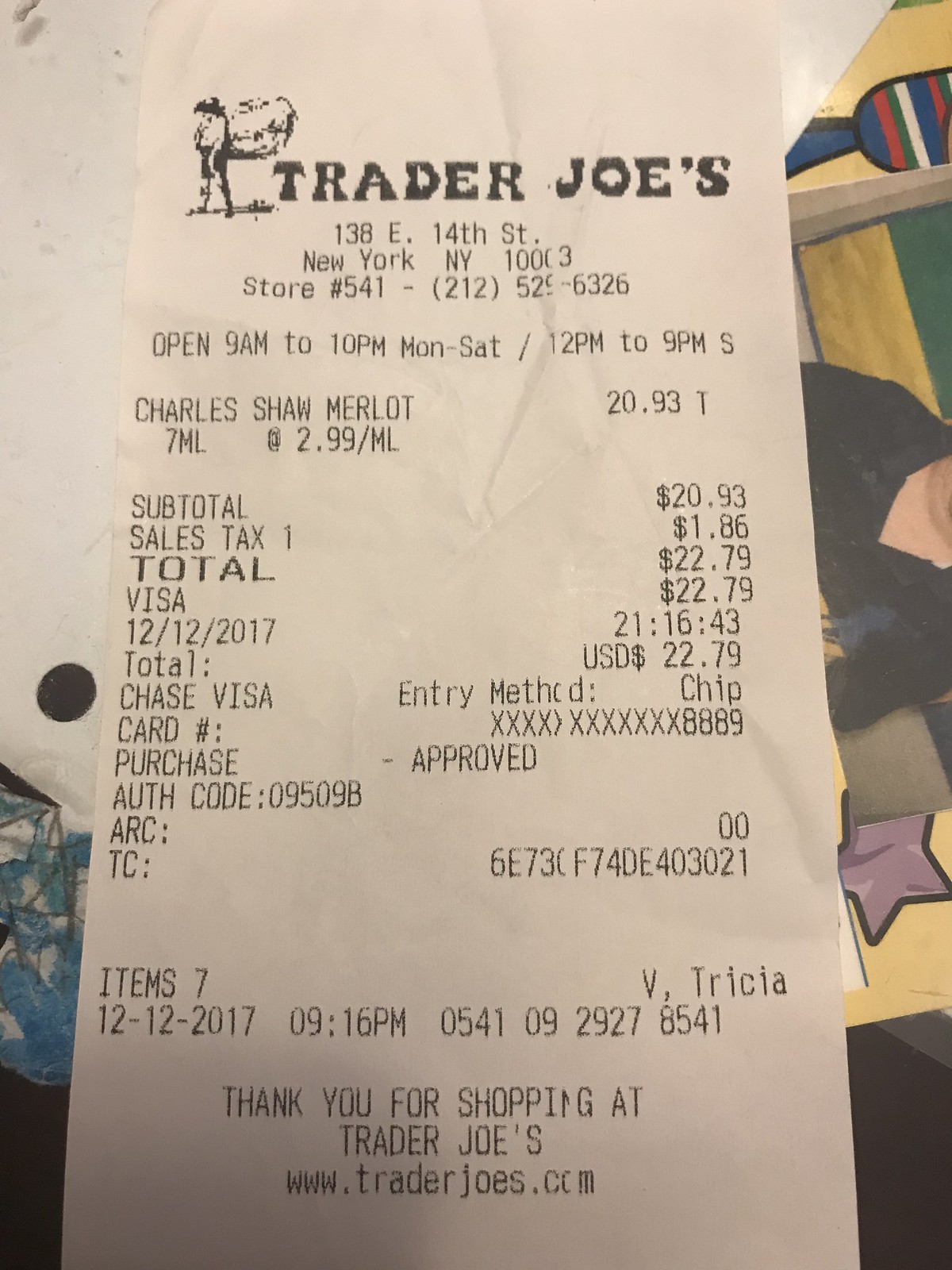This image captures a detailed receipt from Trader Joe's, specifically the one located at 138 East 14th Street, New York, New York, store number 541. The store's contact information is provided, though one digit of the phone number is missing due to a printing issue or the receipt’s age. The store's operating hours are listed as 9 a.m. to 10 p.m. from Monday to Saturday, and 12 p.m. to 9 p.m. on Sunday.

The receipt details the purchase of a bottle of Charles Shaw Marlowe wine, priced at $2.99 for 7 milliliters, totaling $20.93 before tax. With a sales tax of $1.86, the final amount comes to $22.79. The payment was made using a Chase Visa card, and the transaction occurred on December 12, 2017, at 9:16:43 p.m. The receipt includes various authorization details such as the authentication code, ARC, and TC. It records seven items in total, and the cashier or the person who processed the transaction is possibly named Trisha.

The receipt concludes with a thank you message for shopping at Trader Joe’s and the store’s website, www.traderjoes.com.